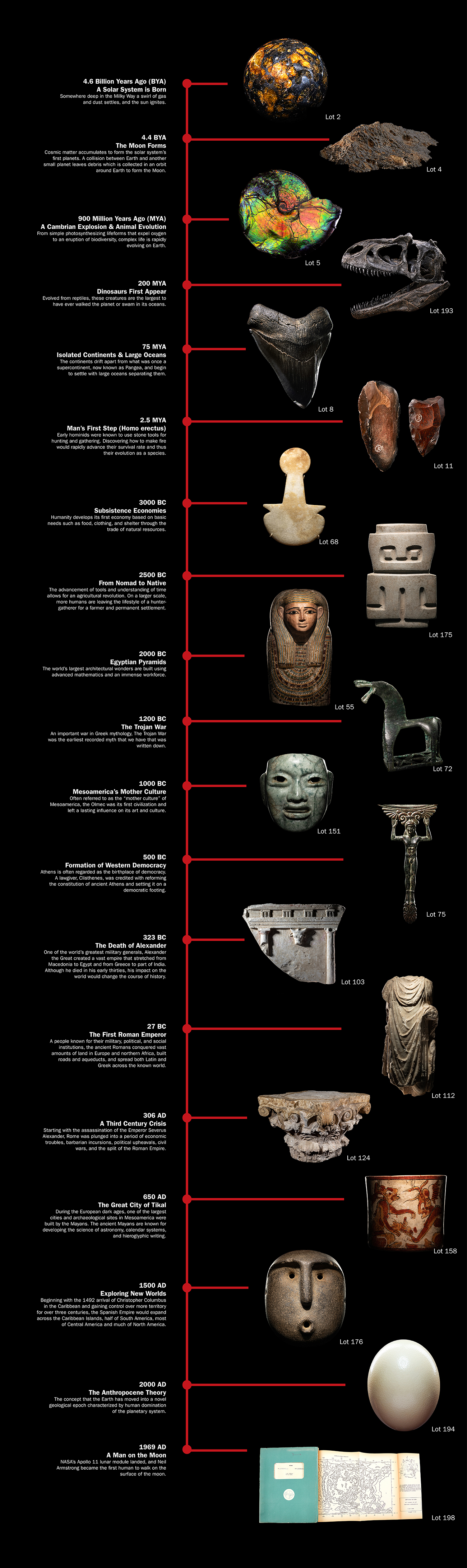The image depicts a vertical timeline with a black background, presenting significant events in Earth's history. At the top, a bold white text reads "4.6 billion years ago (BYA)," marking the birth of the solar system with an illustration of a planet in black, yellow, and gold hues. Directly below, another milestone is marked as "4.4 BYA," detailing the formation of the moon alongside a photo resembling a moon rock.

The timeline continues with a series of events and corresponding images that zigzag down the page from left to right. At "around 541 million years ago (Mya)," a description of the Cambrian explosion, crucial for animal evolution, is illustrated by colorful depictions of early marine life forms. Dinosaurs first appear "around 230 Mya," represented by the skeletal head of a dinosaur.

The sequence progresses through various eras, highlighting significant evolutionary and historical moments, all the way down to "1969 AD," each paired with relevant imagery such as bones, cells, and artifacts. The bottom-most images include a white egg and a map, providing a comprehensive, visual journey from the origins of the solar system to the modern era.